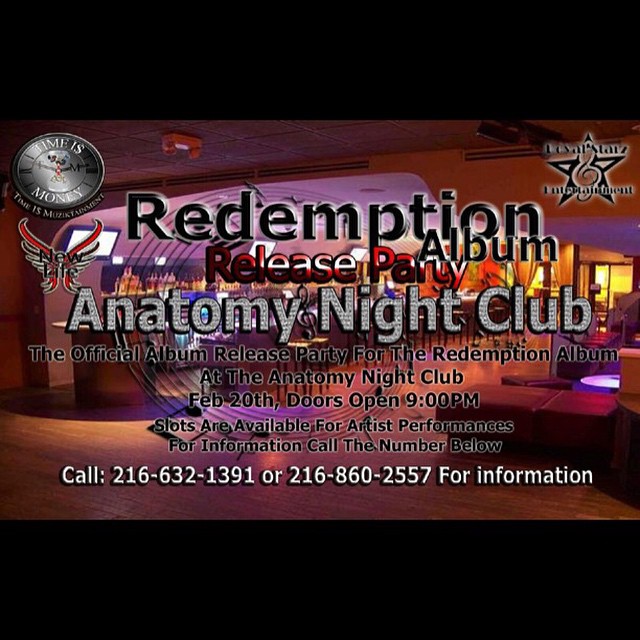The image is a promotional advertisement for a nightclub event titled the "Redemption Album Release Party." The text superimposed on the moody, atmospheric background reads "Redemption Album Release Party" in striking fonts with "Redemption Album" in black and "Release Party" in red. Below this main heading, "Anatomy Nightclub" is displayed in a silver metallic font, reminiscent of a disco ball. Additional text provides further details in black font: "The official album release party for the Redemption album at the Anatomy Nightclub, February 20th, doors open 9 p.m. Slots are available for artist performances. For information call the numbers below." At the bottom, contact numbers are listed in white: "Call 216-632-1391 or 216-860-2557 for information," noting a minor typo with a capitalized "Four." 

The image features a darkly lit room colored in hues of brown, red, gold, and light purple, creating a captivating and lounge-like atmosphere. The layout includes a bar on the left side, barstools in the middle, and additional seating on the right. At the top corners, logos are present: the top left features a grey clock logo with the phrase "Time is Money," and a red eagle logo below it, while the top right showcases a star logo. Black bars frame the top and bottom of the image.